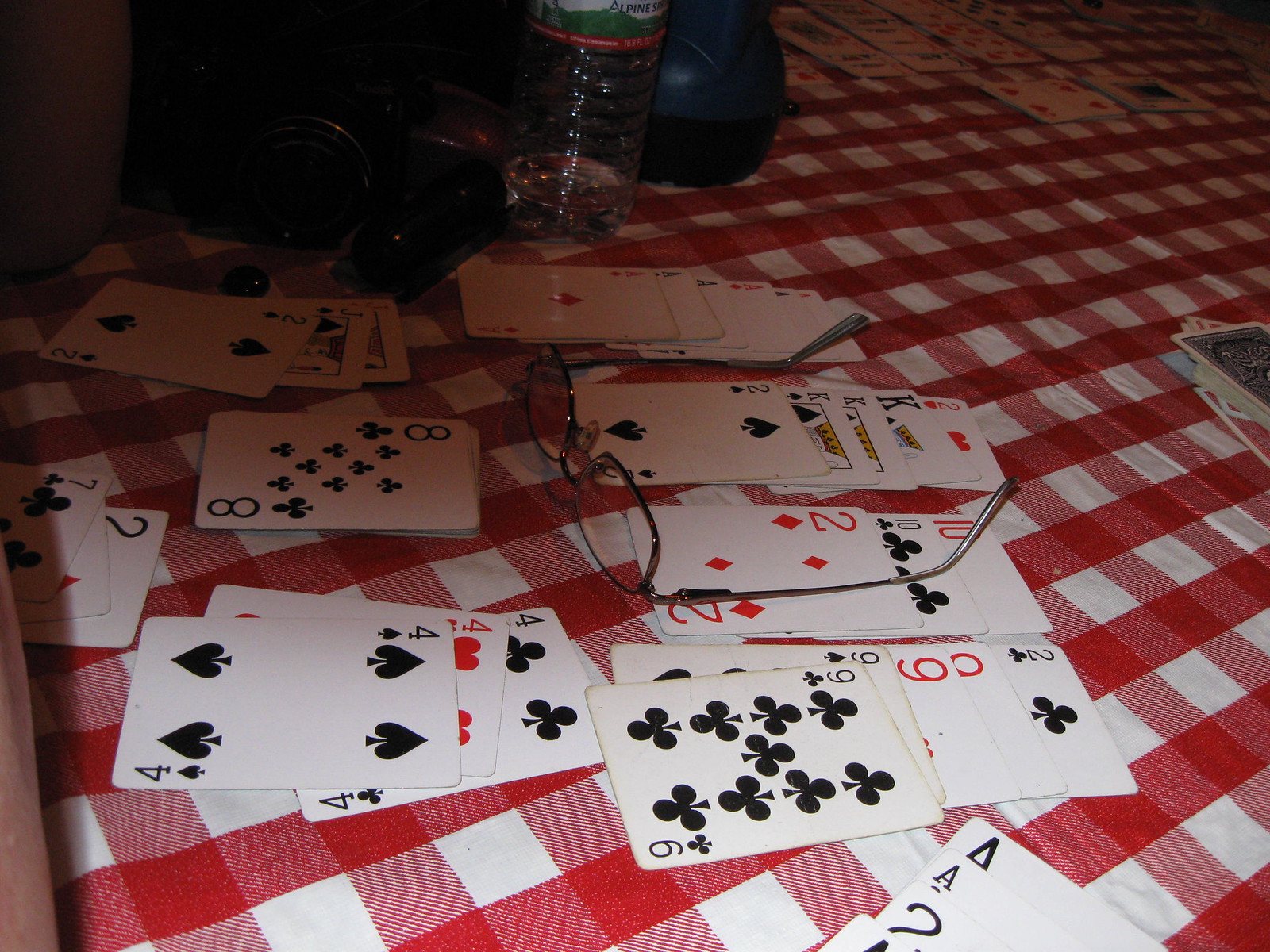A vibrant scene is laid out on a table draped with a classic red and white checkered tablecloth. Centered on the table is an almost empty water bottle, and next to it stands a blue bottle or vase. Nearby, a black object, potentially a camera, lies alongside a small round black item. The table is strewn with playing cards, arranged as if multiple games of solitaire are in progress. A pair of silver-rimmed glasses rests among the cards. One deck of cards features blue backs, while another portion of the deck includes red-backed cards. The face-up cards reveal various suits - clubs, spades, hearts - indicating an active engagement in the game. Despite the absence of people, the scene is lively, suggesting ongoing card games on a peaceful, cozy afternoon.